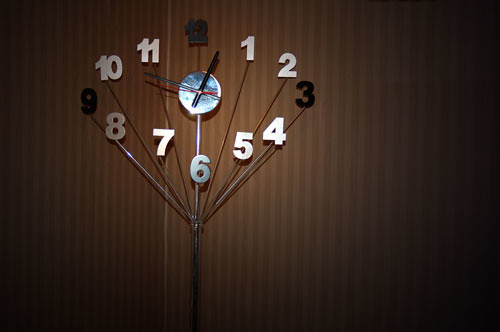The image showcases the interior of a room with a strikingly distinctive ambiance. The focal point is a dark accent wall adorned with sophisticated brown striped wallpaper. The wallpaper features alternating stripes of deep, rich brown and a lighter, contrasting brown, all running vertically up the wall. On the left side of this wall, an eye-catching clock serves as a piece of art and functionality. The clock appears to be crafted from wire, embodying a whimsical, broomstick-like design. The wire rods, gathered centrally, fan outwards like tree branches, with each branch holding a silver metal cutout number, creating a unique, airy frame. The clock's dial is a bold blue circle, punctuated by black hour and minute hands, and a vibrant red second hand, all extending from the center. This unusual and artistic clock adds a quirky, yet elegant touch to the room's overall decor.